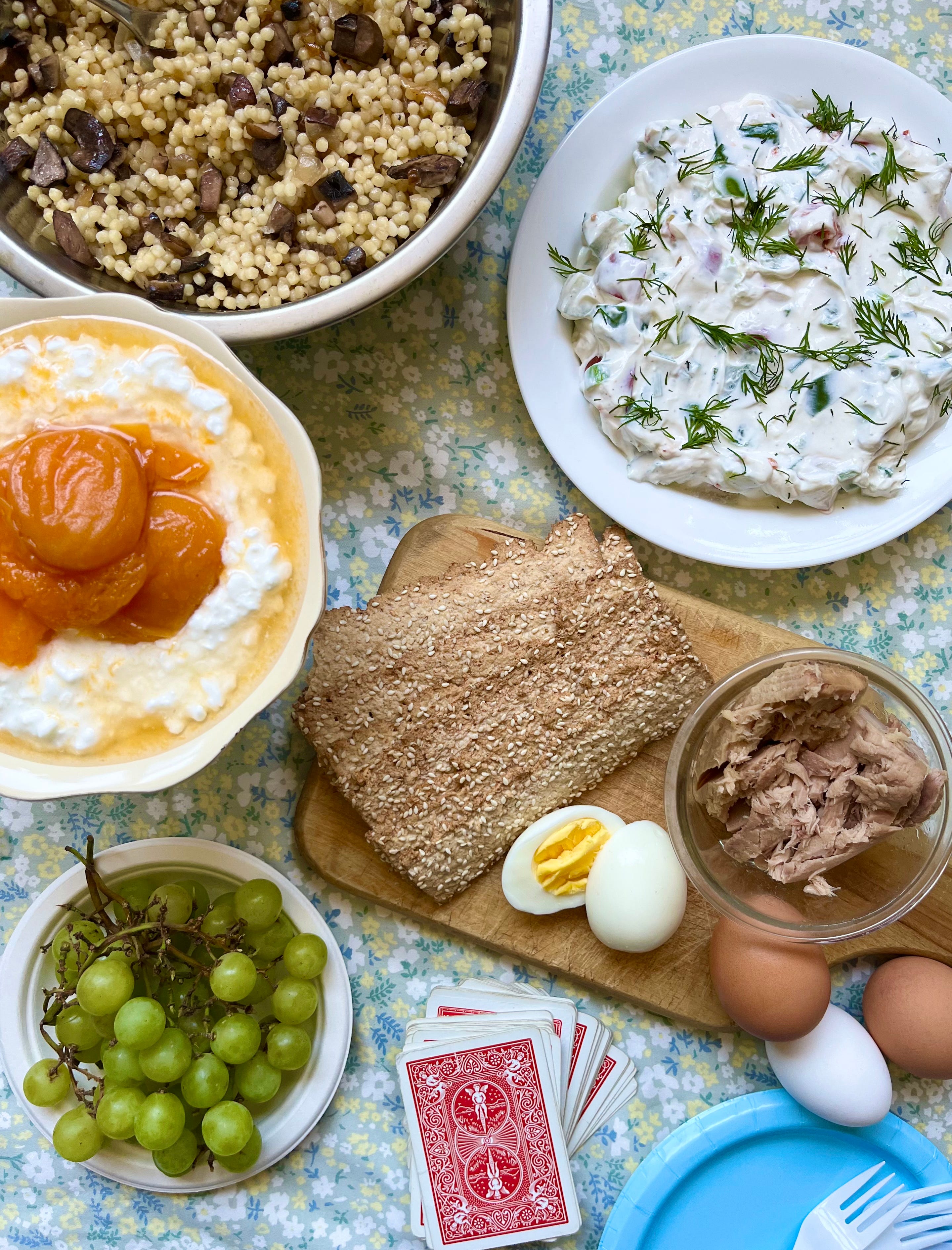A top-down photograph captures a vibrant tablescape, revealing a diverse array of dishes on a light blue tablecloth adorned with white, blue, and yellow floral patterns. Central to the spread is a large bowl of yellow couscous topped with what appears to be either mushrooms or dates. Below, a bowl of green grapes sits on the left. Nearby, a serving of sweet potatoes garnished with marshmallows sits on a white plate, while a creamy dish possibly of mashed potatoes or cottage cheese with herbs or peaches is positioned alongside. 

Toward the right, a large plate holds red potato salad dressed in a thick, mayo-like sauce with dill. Adjacent to it, a wooden board presents long slices of rye bread with seeds, accompanied by a hard-boiled egg cut in half. A small bowl of what seems to be boiled meat and a few whole eggs are scattered around. At the very bottom, a deck of red playing cards is fanned out, near a blue plastic bowl and white plastic forks. The scene is lively, with the dishes offering a kaleidoscope of textures and colors, capturing the essence of a shared, hearty meal.